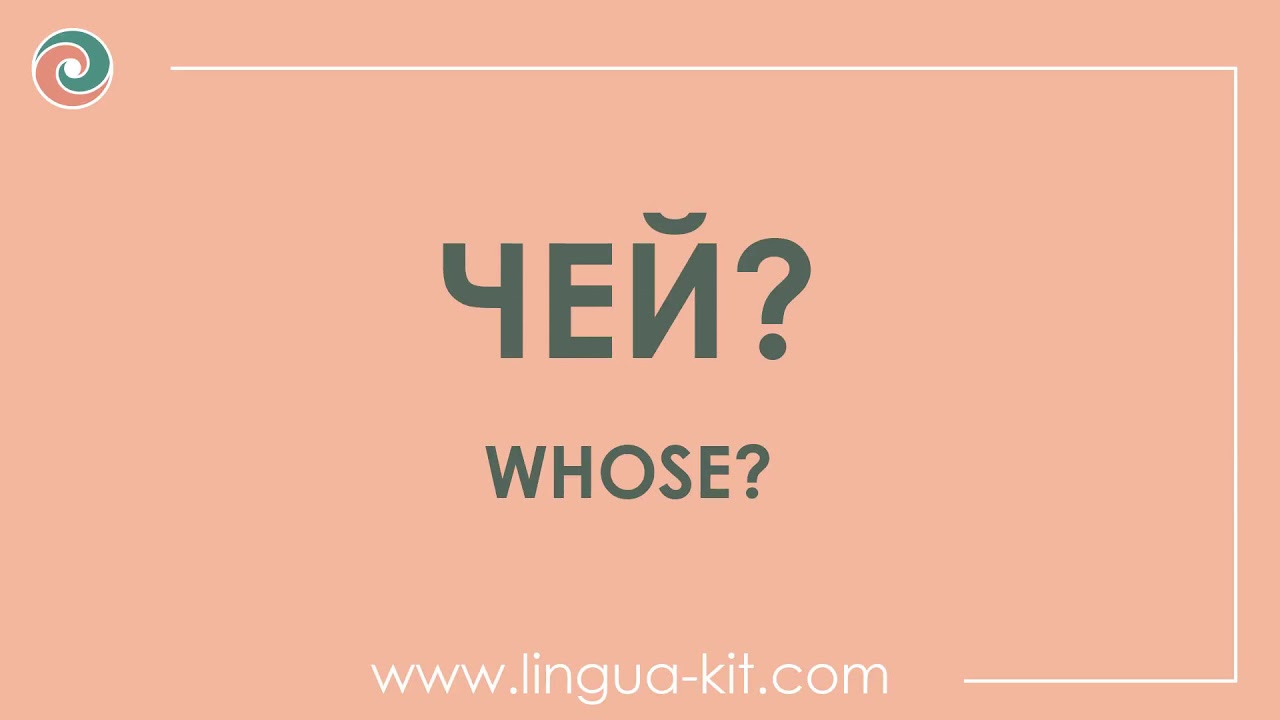The image is a horizontally-oriented rectangle with a peach-colored background, approximately twice as wide as it is tall. In the top left corner is a circular logo featuring green and peach-colored swirls that twist inward toward a white center, all outlined with a thin white line. Extending from the top left corner, a thin white line follows the top border to the right edge, then travels down along the right side and partially along the bottom right corner, serving as a border.

At the center of the image, there is text in an unfamiliar language, styled in gray font. This text includes unique characters such as an inverted, mirrored 'Y' or a character resembling an upside-down lowercase 'H', followed by a capital 'E', a backwards 'N' with an accent, and a question mark. Below this foreign text, the word "who's?" appears in white font. At the very bottom of the image, the URL "www.linguakit.com" is displayed in white.